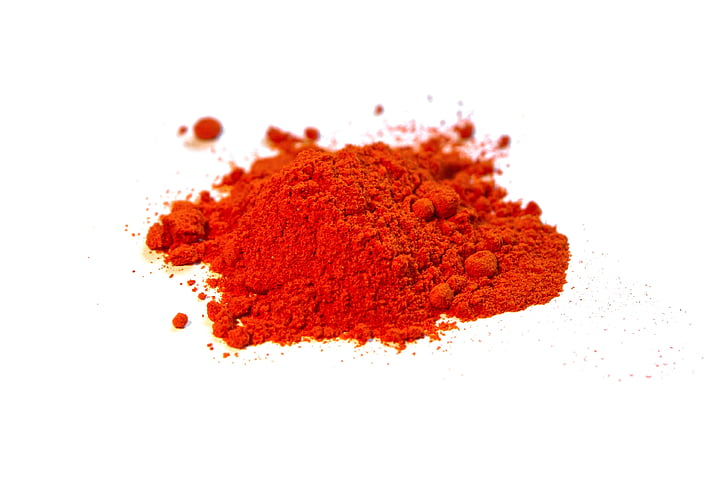A bright, cool-toned red powder, possibly a spice such as paprika or turmeric, is piled up in a large, pyramid-like shape on a pure white surface. The fine consistency of the powder is interrupted by round clumps and small balls, some of which have rolled away from the main pile. These scattered balls and specks create a non-uniform pattern around the base of the mound. The photograph highlights the contrast between the intensely colored powder and the stark white background.